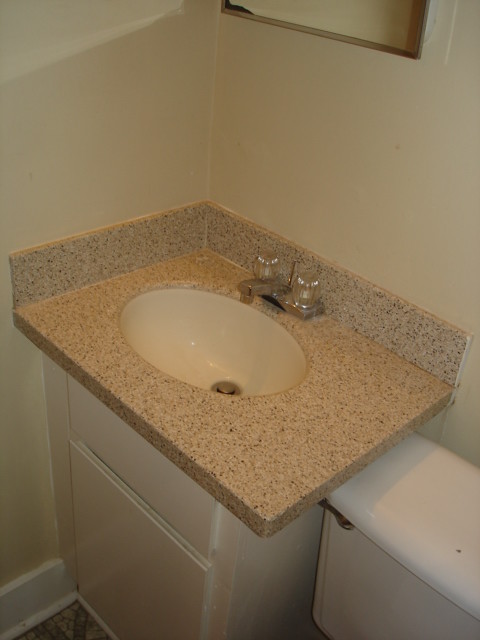This image showcases a small bathroom sink seen from a downward angle. The sink is set within a limited counter space, approximately three inches wide on the left side before meeting the wall, and about six inches on the right. The sink itself is crafted from a gold and brown speckled granite. Despite its age, marked by normal silver tarnishing, the sink features clear plastic knobs.

The sink is mounted on a simple cabinet, consisting of a smaller top drawer and a larger bottom drawer. The walls around the sink are painted beige, accented by white crown molding visible in the upper left corner of the image. Below the sink, a portion of the floor tile is captured, which exhibits a snakeskin-like pattern.

To the right of the sink, the upper part of a white toilet is visible, complete with a silver flush handle.